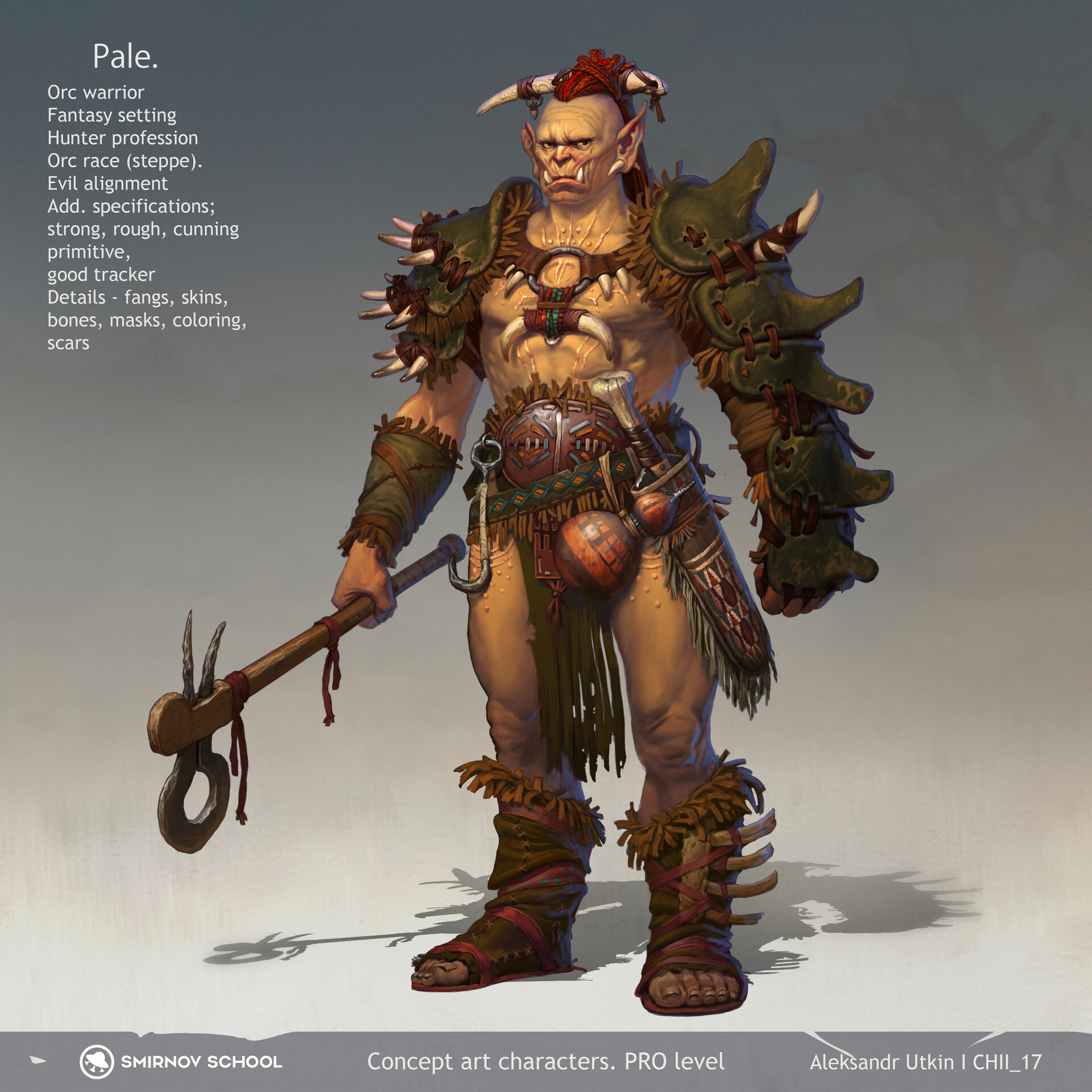The image is a digitally created concept art of a fantasy character, possibly for a game, animation, or graphic novel. Set against a background that transitions from gray to white, the scene showcases a menacing orc warrior. The top left corner contains several descriptive phrases: "Pale Period, Orc Warrior, Fantasy Setting, Hunter Profession, Orc Race, STE, PPE, Evil Alignment, Strong, Rough, Cunning, Primitive, Good Tracker, Details, Fangs, Skins, Bones, Mask, Coloring, Scars." 

The central figure is a large humanoid creature with a muscular build, adorned in a mix of primitive armor made from brown and green materials. The green parts serve as extra padding, secured with large brown threads. The orc's headwear includes red hair in the center and a headband made from what seems to be elephant tusks, leaving the sides of the head bald. The face features pointed ears and menacing fangs protruding from its lower lips. His skin is marked with scars, emphasizing his rugged appearance.

He wears various bones as ornaments, including a necklace with bones. His arms and legs are well-defined, and he has adorned his feet with bearskin boots or leather sandals, fastened with red leather and embellished with bones. The chest is bare except for a band linked to his sleeves, from which another bone is suspended, tied with red and green cloth.

He wields a unique weapon that looks like an axe with a circular blade, and a sword is sheathed at his waist along with a hook-shaped weapon on the other hip. A brown pot hangs from his belt, adding to his primitive and menacing aesthetic. At the bottom of the image, a gray horizontal strip includes the text "Shchernov School, Concept Art Characters, Pro Level, Alexander Ukin, CH 2-2, underscore 17."